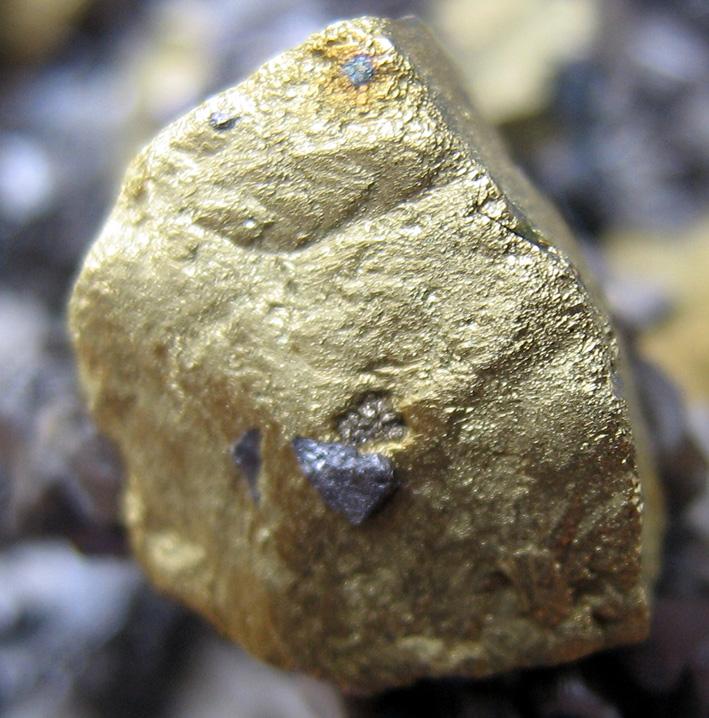This image is a professional, vertically-oriented close-up of a gold-colored rock, prominently centered and occupying most of the frame. The rock appears to have been painted gold, as it features flecks of silver and gray emerging from the gold surface, with hints of rust at the top. The background is entirely blurred, with tones of gray and faint yellow that might suggest other rocks, though they remain indistinct. The lack of text or description adds to the ambiguity of the context. Despite the zoom, possibly making the rock appear larger than it is, its surface details are highlighted, showing a mix of shiny and dulled areas, suggesting it could be pyrite, fool's gold, or simply a painted stone. The stone has a slightly rounded shape and varies in texture and color, with some darker black or brown patches adding to its complex appearance.